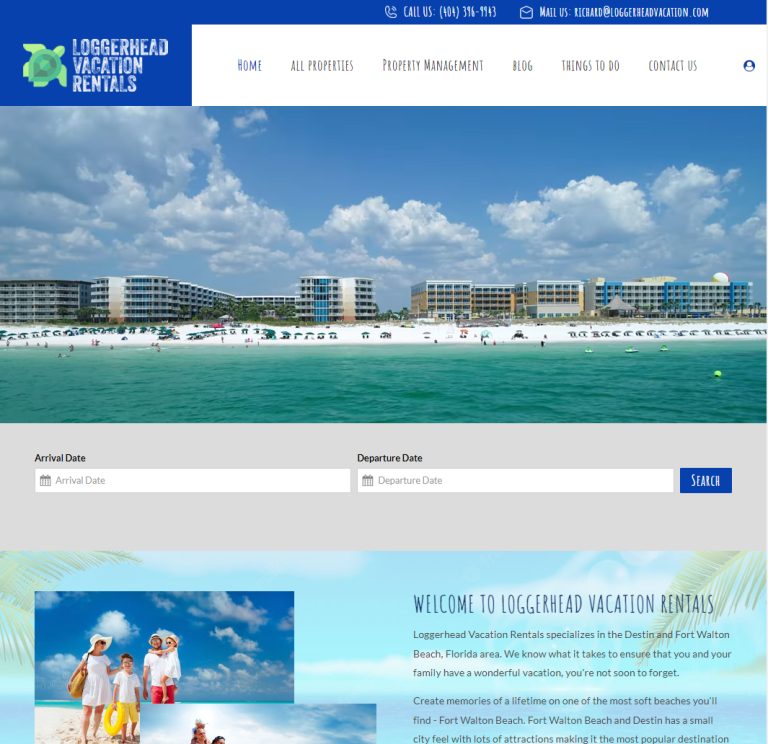The image showcases a vibrant and visually appealing web page themed in shades of blue, green, and white, with accents of light blue. At the top left, a blue banner prominently features a green sea turtle, representing the logo of "Loggerhead Vacation Rentals" in bold white block lettering. Adjacent to the banner, a contact section provides a phone number, "Call Us, 404-396-9543," and an email, "mailusrichard@loggerheadvacation.com."

Beneath this, a white navigation banner displays menu options: Home, All Properties, Property Management, Blog, Things to Do, and Contact Us, facilitating easy navigation through the site. Dominating the page is an expansive photograph of a picturesque beach with pristine white sand and teal green water, accented by a bright blue sky marked with fluffy white clouds. The beach scene is lively with long stretches of buildings lining the shore and beachgoers relaxing under colorful umbrellas.

A search bar, shaded in blue, offers user-friendly inputs for selecting arrival and departure dates. At the bottom of the page, another inviting photograph captures a family enjoying their time on the beach, adding a personal touch and emphasizing the family-friendly nature of the vacation destination.